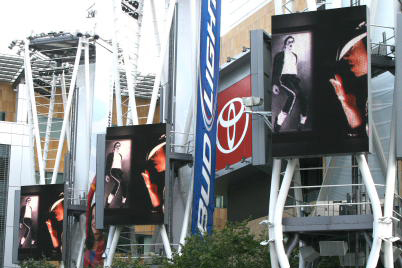This detailed color photograph depicts an outdoor area, possibly the exterior of a stadium or commercial building. Dominating the scene are several billboards and banners. At the bottom of the photograph, you can see the top of some trees. Central to the image are three identical billboards featuring Michael Jackson. Each billboard displays a black and white photograph of Michael Jackson standing on his toes, alongside a side view of him in color, wearing a hat. 

Adjacent to these billboards is a distinctive red sign with the Toyota logo, featuring two linked circles with a smaller circle inside. To the left, a vertical blue banner with white letters prominently displays the words "Bud Light," with "Bud" at the bottom and "Light" extending upward to the top. The billboards and banners are supported by metal poles and fixtures, with probable lighting equipment at the top. The sky visible above is very light blue or white, suggesting a clear or slightly overcast day.